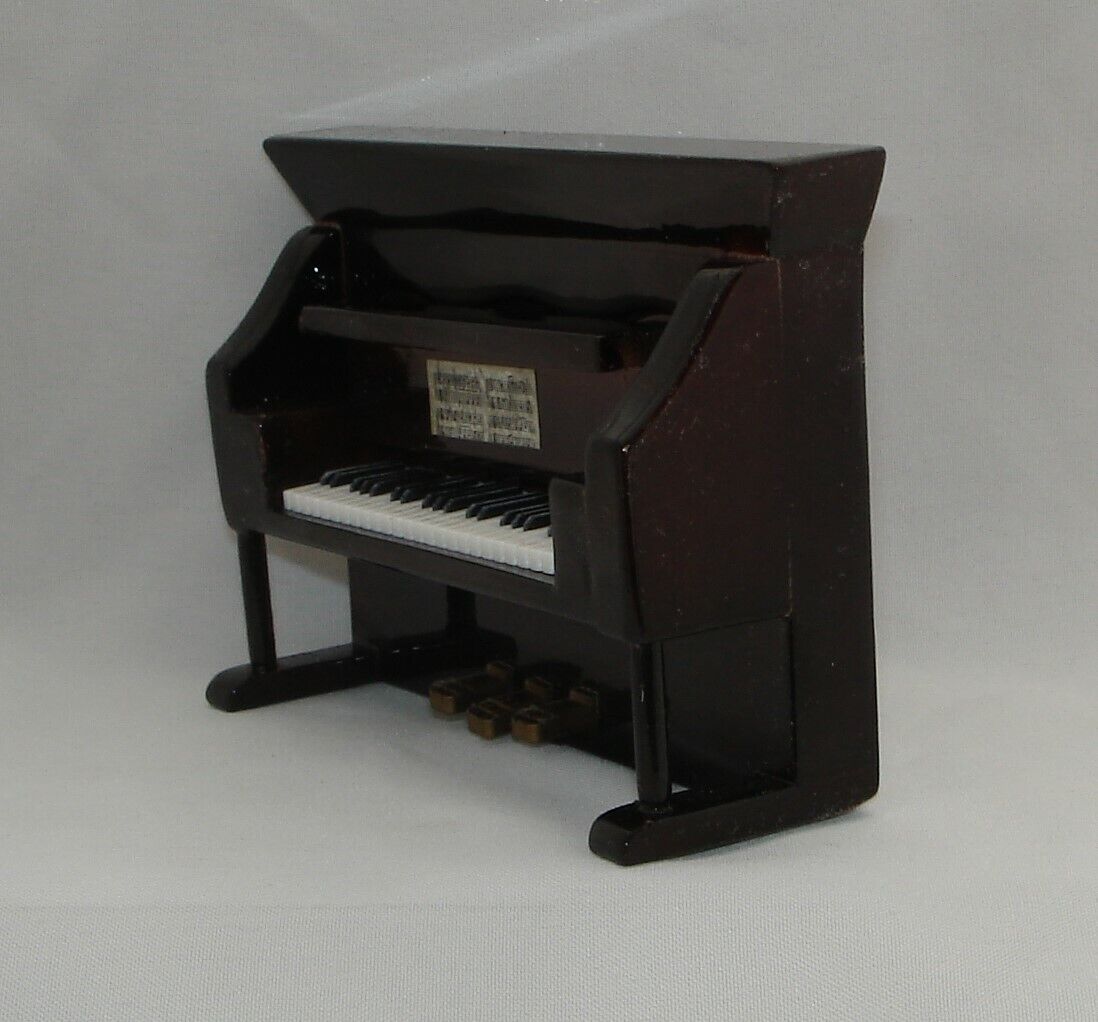The photograph features a close-up of a vintage-styled miniature upright piano ornament, meticulously crafted to resemble a real antique piano. This small-scale model, possibly even fitting for an action figure, showcases finely detailed elements such as tiny individual white and black keys, and three elegant foot pedals below. The piano, made from a dark cherry wood-like material with an overly shiny finish, stands tall and narrow, leaning slightly forward on an off-white cloth background. Above the keys, a miniature sheet music booklet with visible notes adds to the authenticity. The scene is lit with neutral lighting, highlighting the intricate craftsmanship and the piano's prominent position in the image.